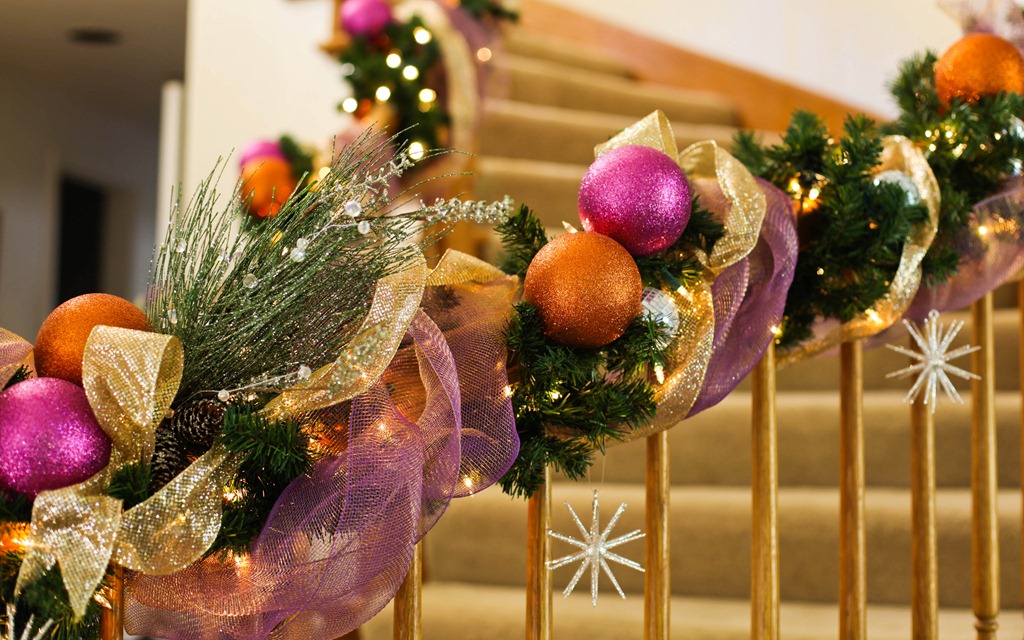This indoor photograph showcases a beautifully adorned spiral staircase, likely within a home. The staircase, carpeted in a brown-beige hue, features light brown, ambery wooden rails. These rails are festively decorated with lush garlands, comprising both spruce and pine elements, intertwining the staircase with holiday spirit. The garlands are further embellished with sparkling warm yellow lights and various decorative elements. Gold and purple ribbons elegantly spiral around the banister, accompanied by clusters of ornaments in vibrant colors such as purple and copper-orange. Silver, glittery snowflake ornaments dangle intermittently from the rail, adding a touch of winter charm. The intricate decor, including what appears to be disco ball-styled ornaments, enhances the festive atmosphere, making the staircase a captivating focal point of the holiday décor.